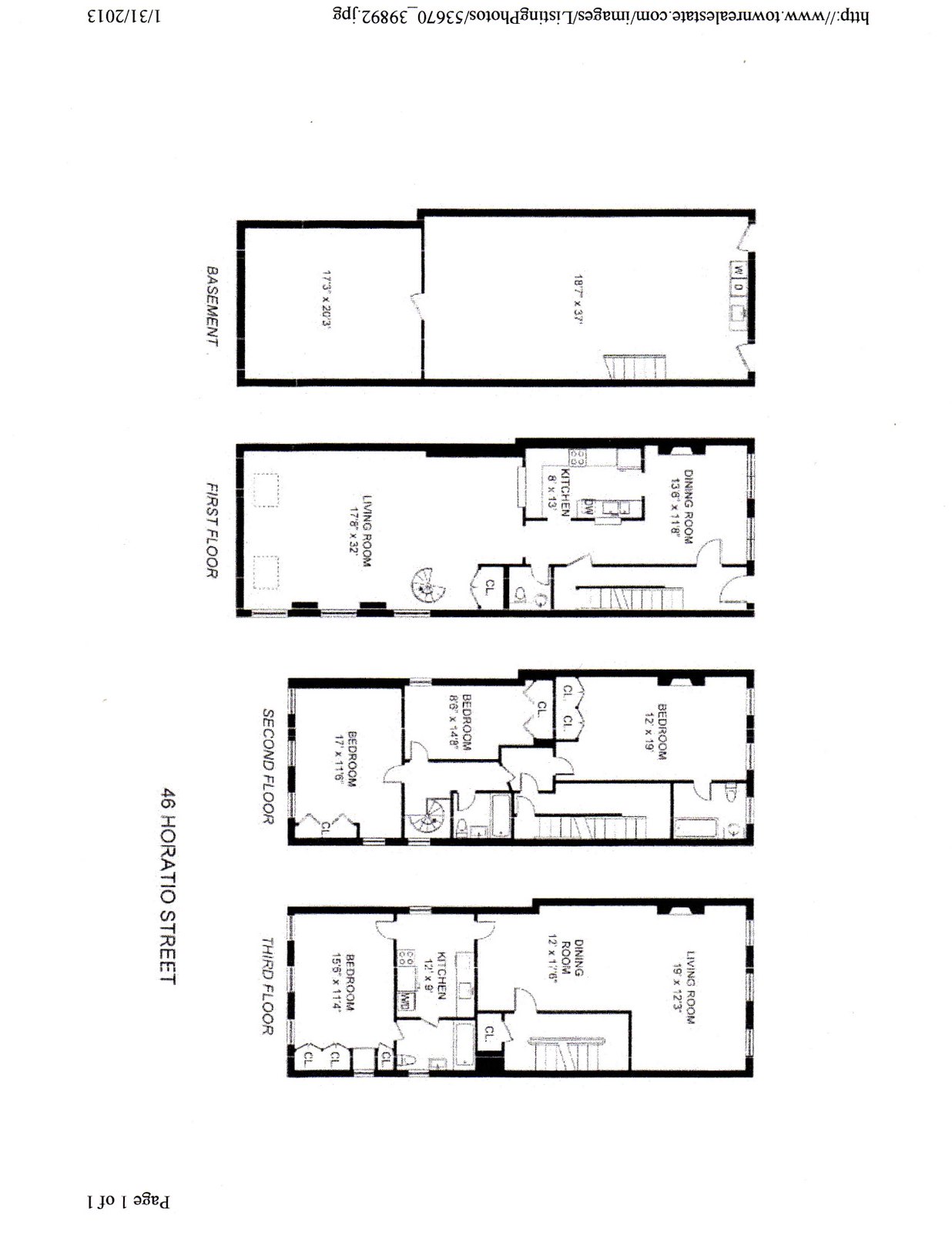This image is a detailed floor plan depicting four levels of a house. From left to right, the plans are labeled "Basement," "First Floor," "Second Floor," and "Third Floor" at the bottom of each section. 

**Basement Plan (far left):**
- Positioned at the bottom, the plan features vertically aligned letters spelling "Basement" from top to bottom, angled towards the right.
- There is a thick black border outlining the basement's perimeter. This border starts at the top, descends and then stretches horizontally across the page with minor vertical deviations.
- Within the black border, there are several openings and fixtures. These openings are positioned sporadically along the border, with small line segments and diagrams indicating various structural elements.

**First Floor Plan (second from left):**
- Situated directly above the basement plan with the label "First Floor."
- The plan features multiple large openings divided by pairs of thick black lines, suggesting doorways or passageways.
- The outline of the floor comprises thick black lines that encircle the floor’s structure. Intermittent smaller openings and small black line segments are indicated throughout, marking possible windows or additional doorways.

**Second Floor Plan (second from right):**
- This level is smaller compared to the basement and first floor.
- The black outline starts from the top left, runs horizontally with small openings interspersed before continuing across the top. The outline then extends vertically, dips down slightly, and completes the perimeter with alternating openings and black segments.
- The layout within includes larger openings, bordered sections, indicating probable staircases or key room transitions. Various designs inside likely depict closets and other small spaces.

**Third Floor Plan (far right):**
- This plan mirrors the second floor closely but with varied room placements.
- The plan repeats the structure of the second floor with black borders, multiple openings, and interior markings for closets and room layouts.

Each floor plan is distinctly labeled and outlined with thick black borders, presenting detailed structural layouts, including spaces for rooms, openings for doors, windows, and other fixtures.